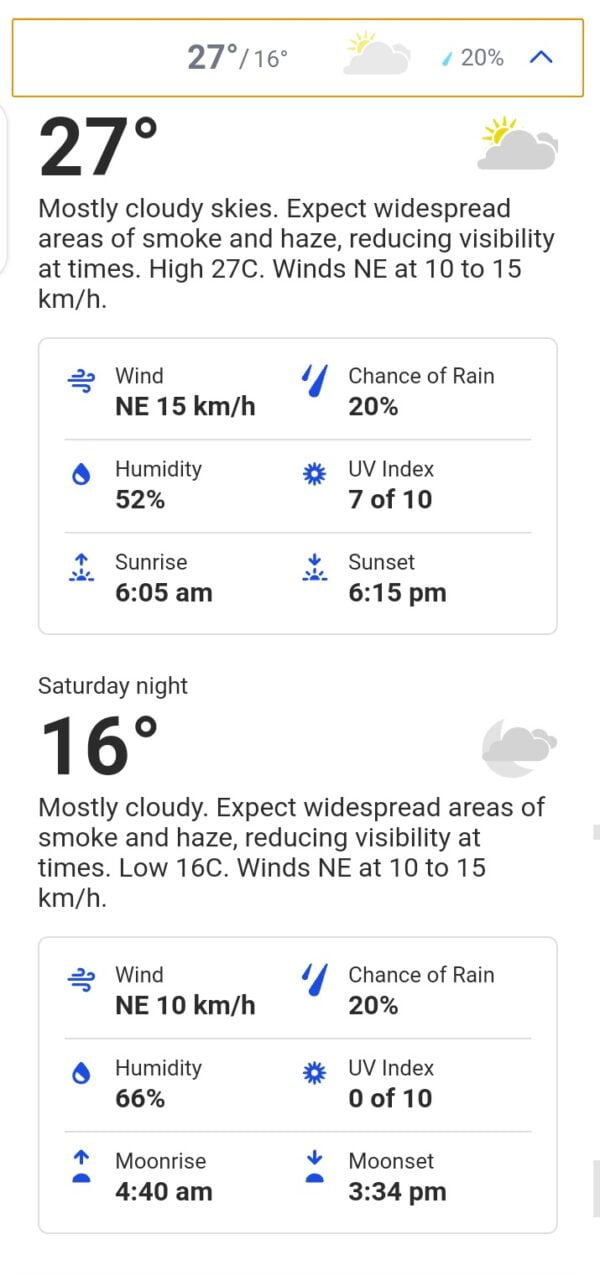The image displays a weather app, though due to the clipped user interface, it is unclear whether it is from an iPhone or Android device. The app screenshot appears to depict the forecast and current weather conditions.

At the top of the screen, there is a rectangular section outlined with a yellow border and a white background. This section likely shows today's forecast, indicating high and low temperatures of 27°C and 16°C, respectively. An icon showing the sun partially obscured by a cloud, alongside the text "20%" and an image of a raindrop, suggests a 20% chance of rain.

Below this section are the current weather conditions. Prominently displayed is the temperature 27°C, coupled with a larger version of the sun-behind-cloud icon. The text notes that the weather is mostly cloudy with widespread smoke and haze, which is expected to reduce visibility. Other details include a high of 27°C, wind speeds from the northeast at 10-15 km/h, 52% humidity, sunrise at 6:05 AM, sunset at 6:15 PM, a UV index of 7 out of 10, and a 20% chance of rain.

Further down, the data switches to the evening forecast, presumed to be for Saturday night. The expected low temperature is 16°C with an icon depicting the moon partly covered by a cloud. The description mirrors earlier conditions, stating mostly cloudy skies with widespread smoke and haze. This confirms the consistency of the weather throughout the day.